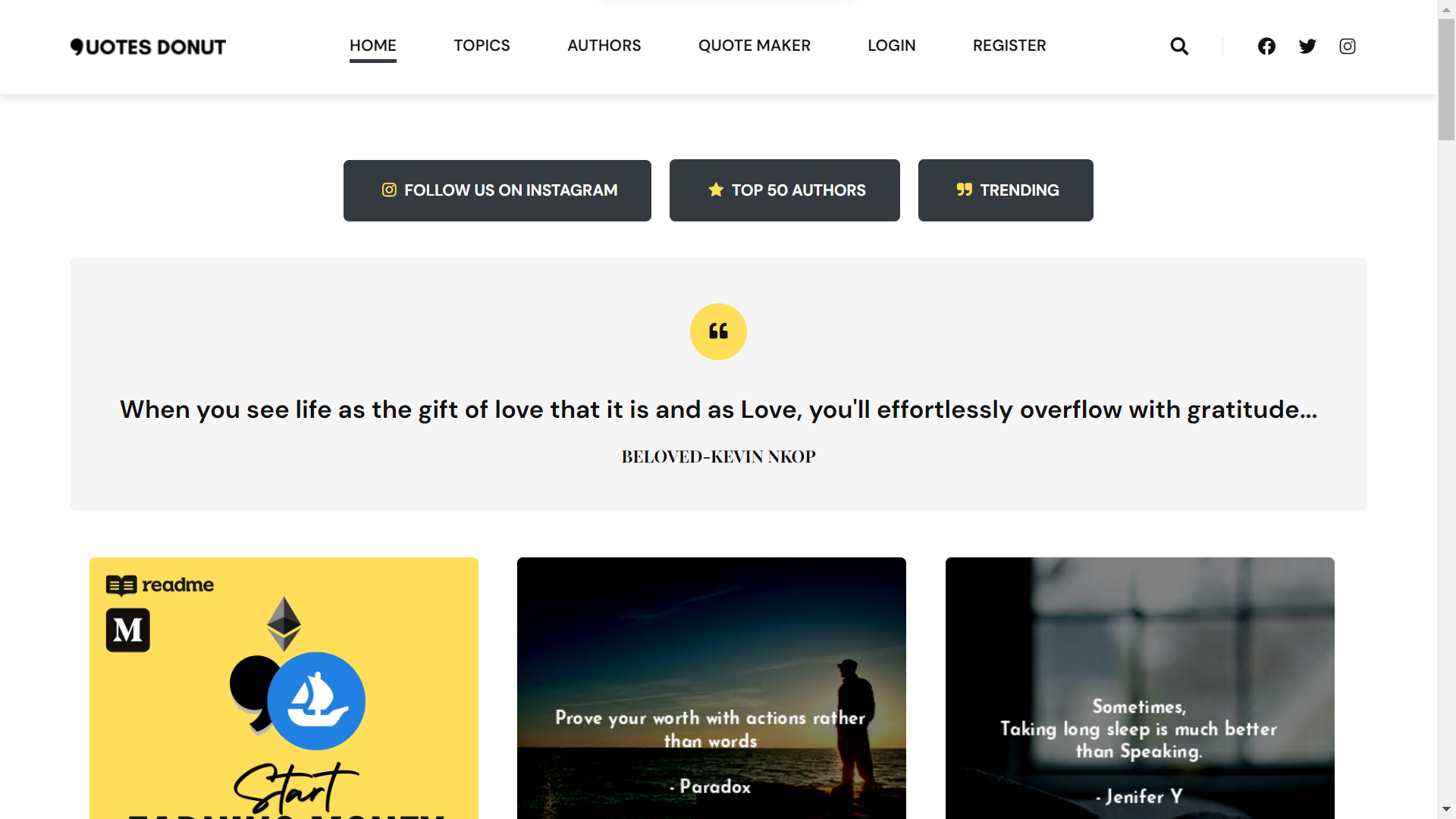This is a screenshot of the Quotes Donut website. The navigation bar at the top features the site name "Quotes Donut" prominently. Following the site name, the navigation menu includes links labeled "Home," "Topics," "Authors," "Quote Maker," "Login," and "Register." An underline beneath "Home" indicates the currently selected page. On the right side of the navigation bar, there are icons for search, represented by a magnifying glass, as well as icons for Facebook, Twitter, and Instagram.

Directly below the navigation bar, centered on the page, there are three prominent buttons labeled "Follow Us on Instagram," "Top 50 Authors," and "Trending." Beneath these buttons, there is a notable graphic: a yellow circle enclosing quotation marks. Below this graphic, a motivational quote reads, "When you see life as a gift of love, that it is, and as love, you'll effortlessly overflow with gratitude," attributed to "Beloved. Kevin," though the text is slightly unclear.

Further down the page, there are three horizontally oriented boxes. The first box on the left is yellow and includes the text "Read Me" alongside an icon of an open book. Next to this, a white "M" is set within a black square. The second, central box contains an image of a man gazing into the distance with the quote "Prove Your Worth in Actions Rather Than Words," attributed to "Paradox." The third box features an icon of a white ship inside a circular emblem.